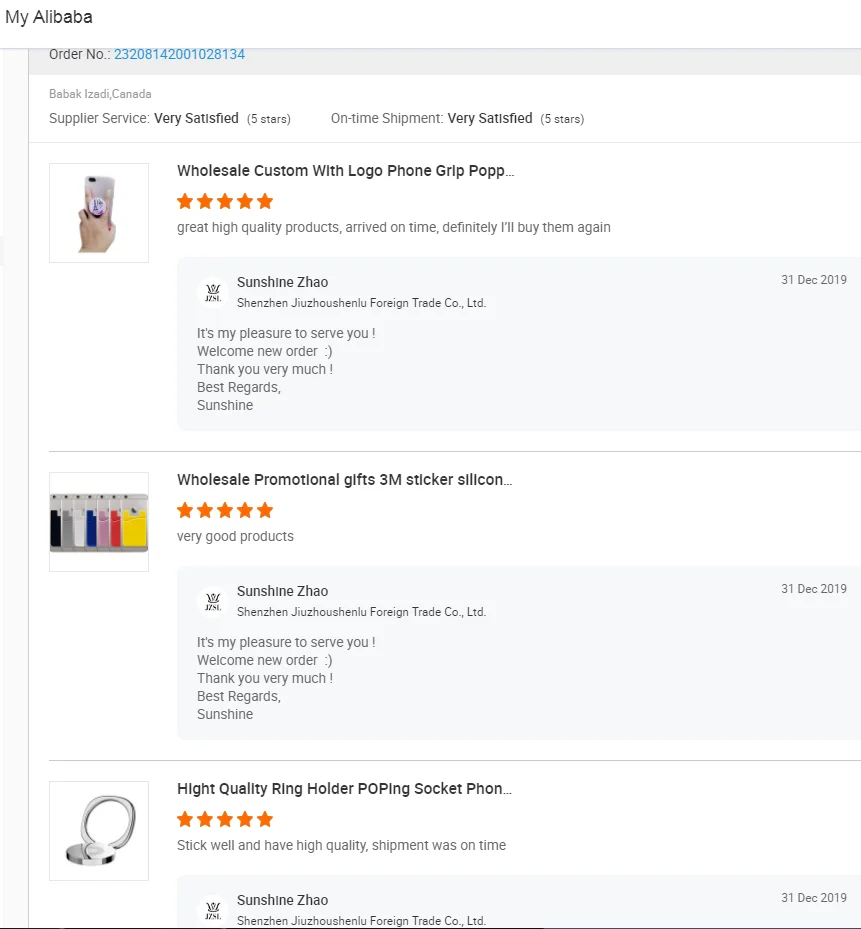In this screenshot from an Alibaba account, the user's order details and ratings are displayed. At the top, a white bar stretches across the screen with "My Alibaba" written in black on the upper left corner. Below, a gray bar shows "Order Number" followed by a sequence of blue, clickable numbers. The shipping information beneath reveals "Canada, Babak Izadi, Canada," though it remains unclear whether this address belongs to the sender or the recipient.

The user has provided ratings and feedback for three products. The first product is a "Wholesale Custom with Logo Phone Grip Pop," which received a five-star rating. The buyer's review states, "Great high-quality products, arrived on time, definitely I'll buy them again." The supplier, Sunshine Zhao, responded with, "It's my pleasure to serve you, welcome new order, thank you very much, best regards Sunshine."

Additionally, two more products were rated: "Wholesale Promotional Gifts 3M Sticker Silicone" and "High Quality Ring Holder Pop Socket Phone," both of which also received five stars. The buyer commented that these were "good products." Supplier service and on-time shipment for all orders were rated as "very satisfied," with each receiving five stars.